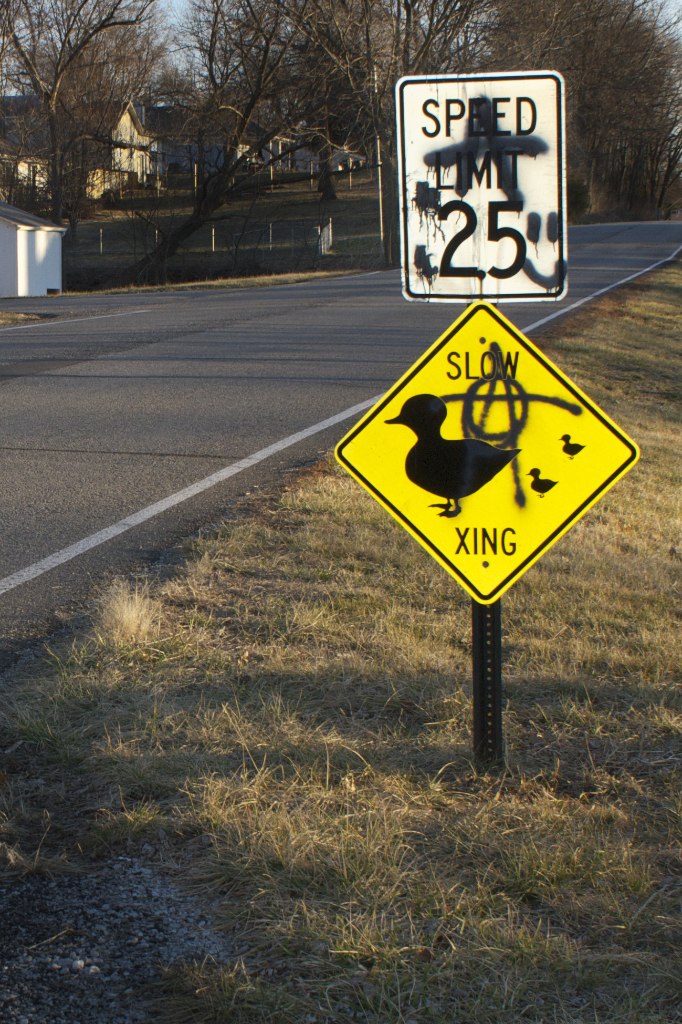A detailed photograph captures a scene of two signboards mounted on a single black pole riddled with small holes, situated beside a diagonally extending gray asphalt road with a white painted stripe along its edge. The pole is embedded in a yellowish-brown grassy patch. The upper sign, a white speed limit sign with black text reading "Speed Limit 25," is marred by graffiti, including an anarchy symbol. Below it, a vibrant yellow diamond-shaped sign, edged in black, displays the word "SLOW" above an image of ducks and the abbreviation "XING." This second sign also bears graffiti. The road occupies the left part of the image, revealing a series of trees and a white building in the background. The dry, predominantly brown grass contrasts with the road's blackish-gray asphalt, accented by its crisp white lines, highlighting the outdoor setting in broad daylight.